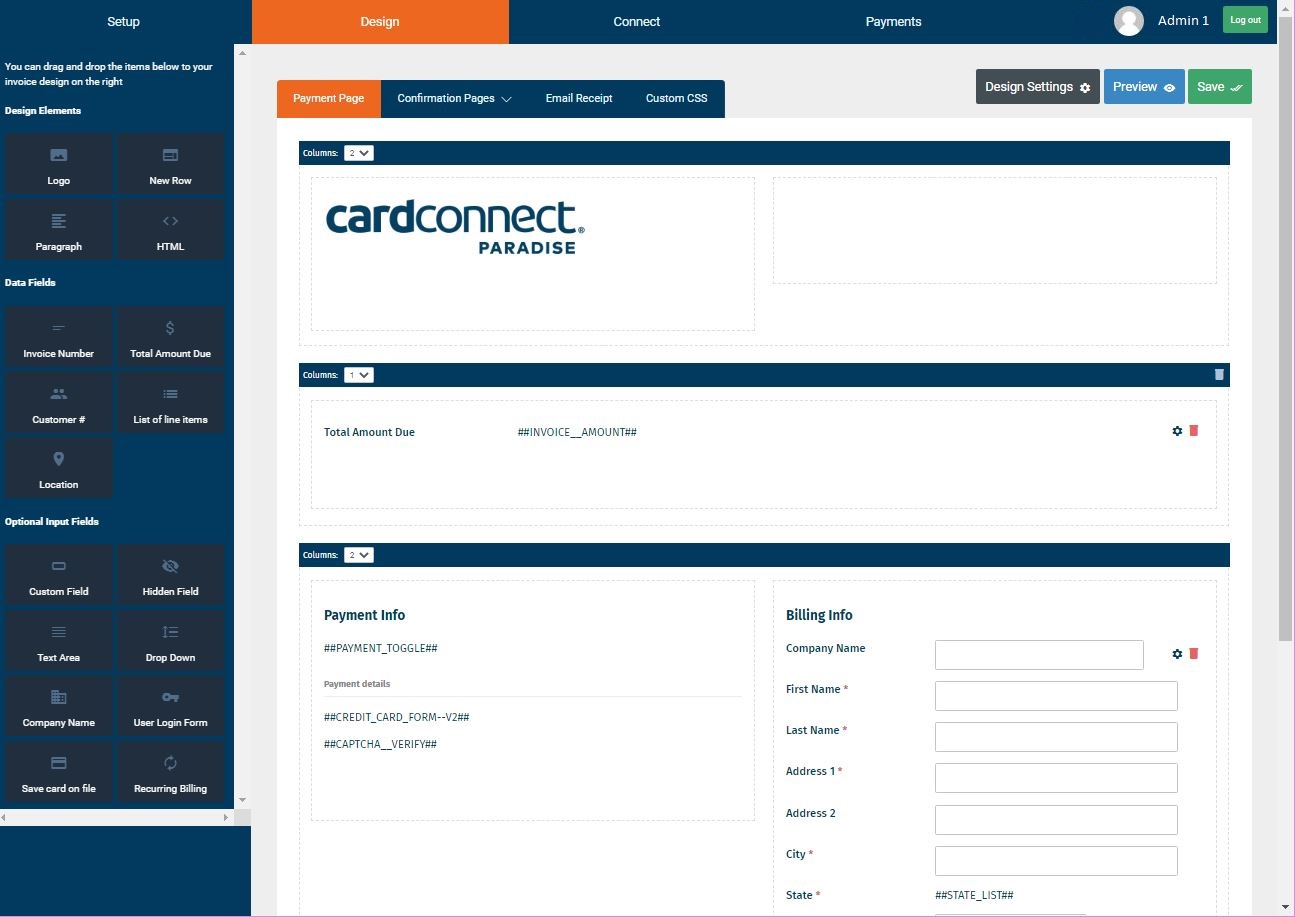The image appears to be a screenshot from a website, possibly related to web design or e-commerce setup. The interface contains a navigation menu at the top with the following tabs from left to right: "Setup" (white text on a blue background), "Design" (white text on an orange background, indicating that this option is currently selected), "Connect" (white text on a blue background), "Payments" (white text on a blue background), and a user icon with the name "admin1" displayed next to it. There is also a green "Log Out" button next to the user name.

The layout is divided into two sections: the left side, which has a menu listing various options such as "Design," "Classes," "Data Fields," and "Optional Input Fields." The right side displays content related to the selected option. Here, it shows headings like "Payment Page," "Confirmation Page," "Email Receipt," and "Custom CSS." Below these headings, there are three buttons: "Design Settings" (gray), "Preview" (blue), and "Save" (green).

Additionally, there is a bar labeled "Kit Card Connect Paradise" below the buttons. Further down, you see sections for "Total Amount Due" and input fields for "Payment Info" and "Billing Info," presumably for processing transactions.